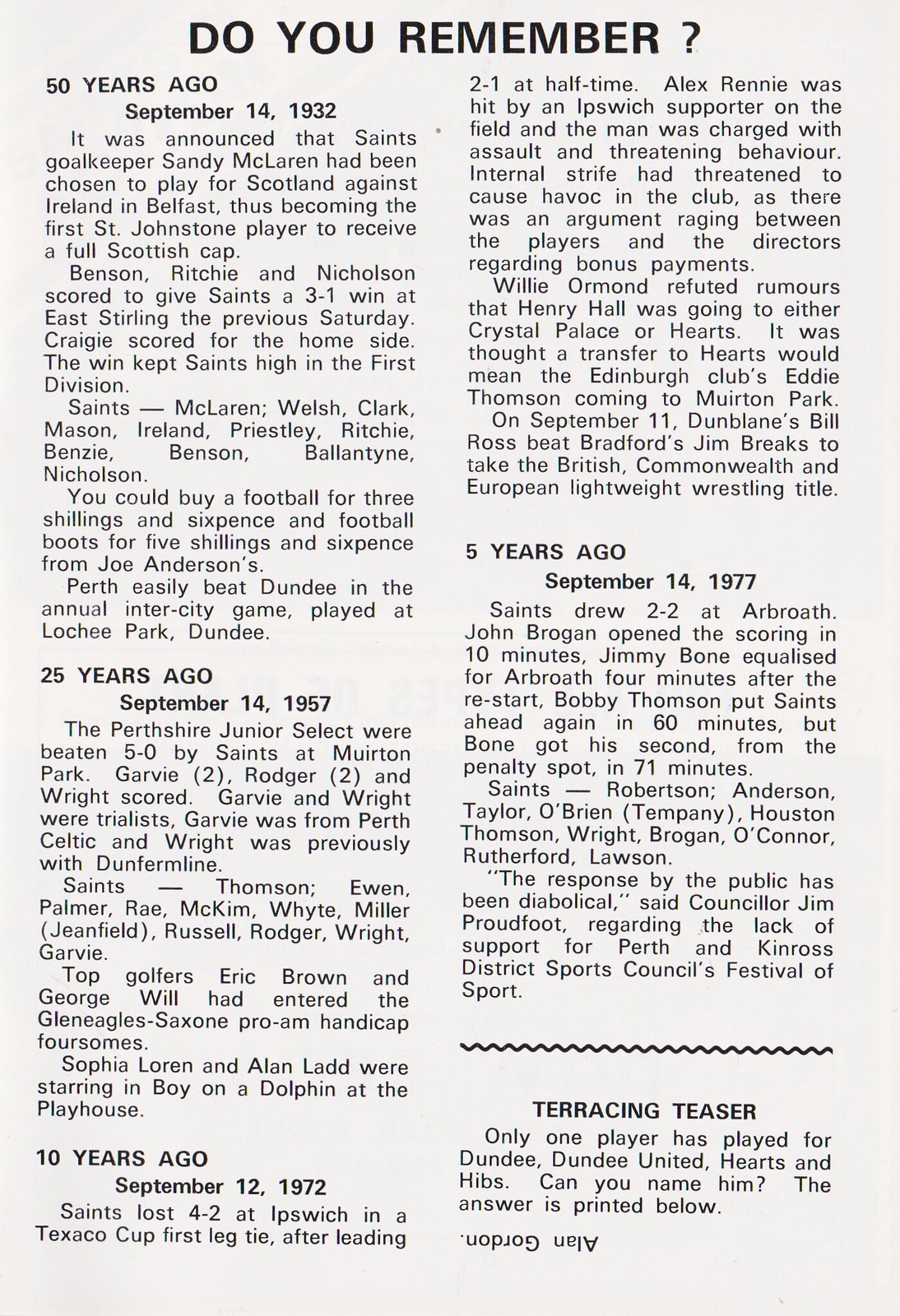A nostalgic newspaper clipping features the title "Do You Remember?" prominently at the top, initiating a dive into soccer history spanning several decades. The clipping is divided into two columns filled with text, recounting significant events. Highlighted prominently is the 50th anniversary on September 14th, 1932, when Saints goalkeeper Sandy McLaren was announced to play for Scotland against Ireland in Belfast, marking him as the first St. Johnstone player to receive a full British cap. Another notable mention is from 25 years ago, on September 14th, 1957, where the Perthshire Junior Selects were defeated 5-0 by the Saints at Mutton Park, with goals from Galby (2), Roger (2), and Wright. Galby, from Perth Celtic, and Wright, previously from Durham, were trialists. Additionally, the column includes mentions of events from 10 years ago (September 12th, 1972) and 5 years ago (September 14th, 1977), as well as a trivia section featuring a teaser on which player has played for Dundee, Dundee United, Hearts, and Hibs, with the answer revealed as Alan Gordon. The imagery reflects a rich history of local soccer, celebrating both extraordinary and everyday achievements.